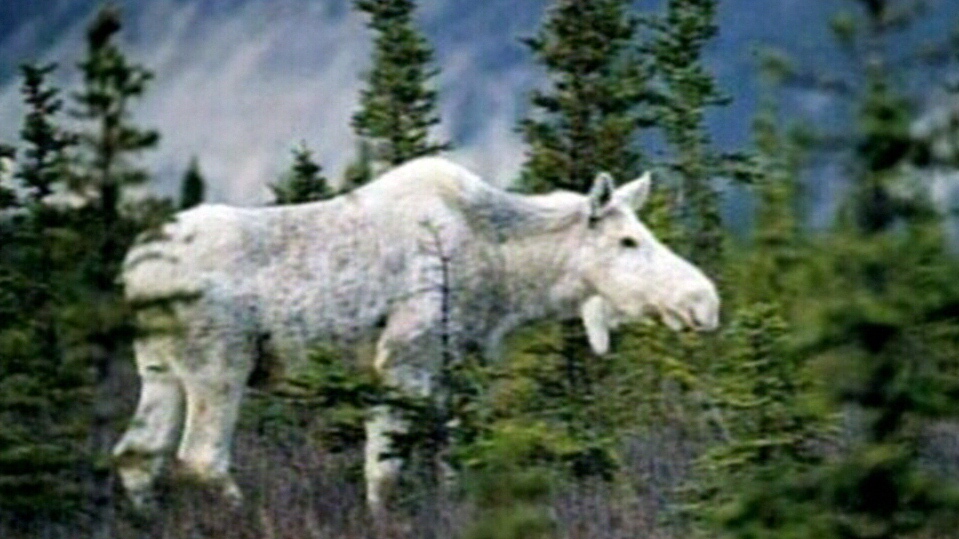The photograph portrays a large, white moose standing in the midst of a dense forest of tall green pine trees. The moose, appearing almost albino with its pure white fur and slight speckling of dark colors, is centrally placed in the image and shown in profile, with its head pointing toward the right. Its distinctive features include the absence of antlers, perked white ears, and a notable hump slightly above its shoulder level. The moose stands in a grassy area filled with grayish weeds and vegetation, while the background reveals a bright blue sky adorned with wispy white clouds. The image, however, seems to be of low quality, characterized by significant compression artifacts and blurriness, particularly at the bottom and on the right-hand side, suggesting it may have been generated by artificial intelligence. Despite these imperfections, the photograph captures the serene beauty of this majestic creature in its natural habitat.